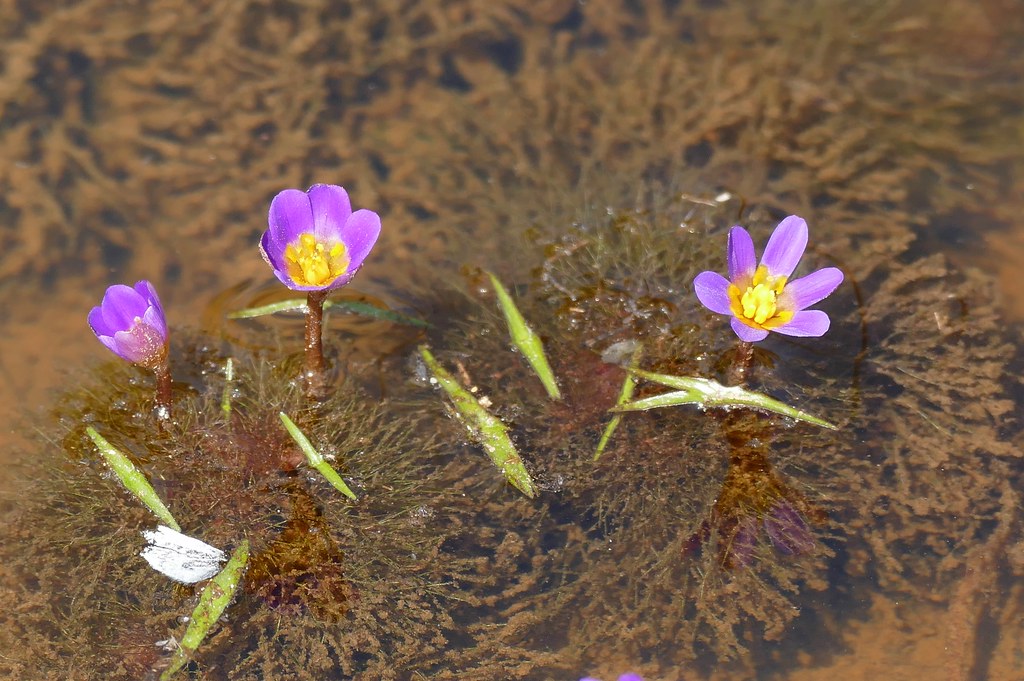In a shallow, underwater setting, a fascinating image reveals a cluster of unique aquatic plants. The background features stringy, brown, thread-like vegetation, creating an intricate underwater tapestry. Emerging from this submerged environment are three captivating flowers, standing out prominently. These flowers, with their delicate purple petals, transform as they rise above the water's surface, showcasing vibrant yellow centers. The petals display a gradient of color, transitioning from lavender pink near the edges to a richer purple hue. At the heart of each bloom, distinct yellow stamens and anthers catch the light. Surrounding the flowers are hints of green stems and leaves, suggesting a rich, underlying growth that supports these remarkable blooms. The scene is framed by a thin layer of water, accentuating the flowers' delicate beauty and the moss-like growth below. This captivating composition highlights the resilience and allure of these underwater blooms.